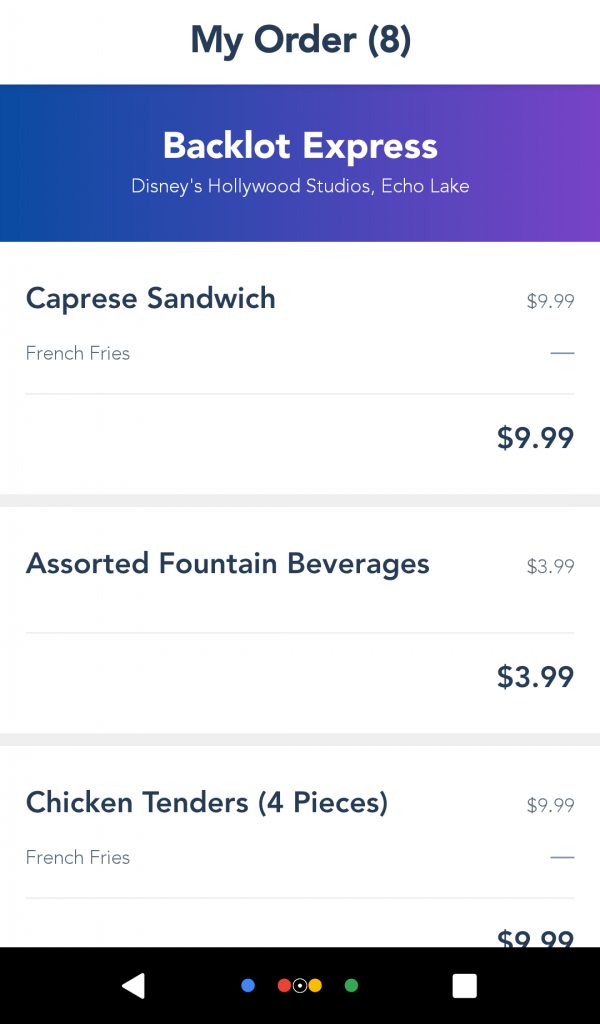The image depicts a smartphone screen displaying an order summary on a user's device. At the bottom of the screen, there is a black ribbon featuring the back, home, and refresh buttons. 

At the top of the page, "My Order (8)" is prominently displayed in bold, navy blue text. Below this, a horizontal rectangular box with a purple background contains the white, bold text "Backlot Express." Just beneath, in smaller white text, it reads "Disney's Hollywood Studios, Echo Lake."

Further down, "Caprese Sandwich" is written in navy blue text, with the price "$9.99" in light gray to its right. Below this item, "French fries" is listed in light gray text, with a placeholder line for the price. The subtotal "Total: $9.99" is shown in bold navy blue text.

Lastly, "Assorted Fountain Beverages" is displayed in bold navy blue text, with its price "$3.99" also in bold text.